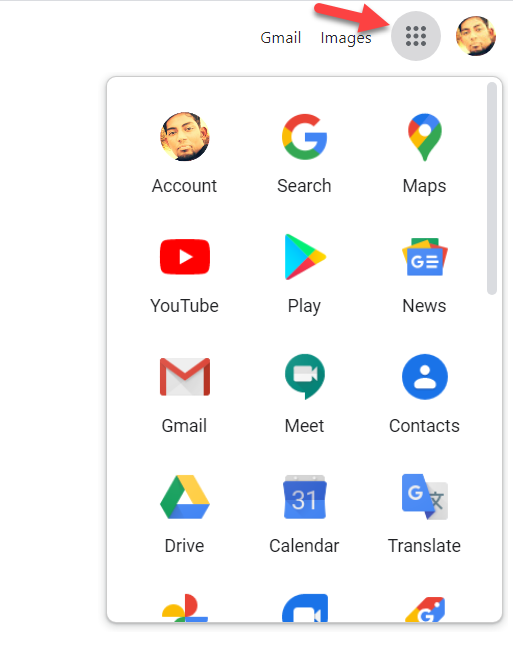This image captures a screenshot of several Google application icons. At the top, it says "Gmail" and "Images," alongside a red arrow pointing at what appears to be a tabs bar or an icon menu option. A profile picture depicting the user is visible in a circular frame. Below, an array of Google service icons is displayed, including Account, Search, Maps, YouTube, Play, News, Gmail, Meet, Contacts, Drive, Calendar, Translate, Photos, and Duo. One additional icon, partially visible and resembling a Google price tag, indicates another Google service.